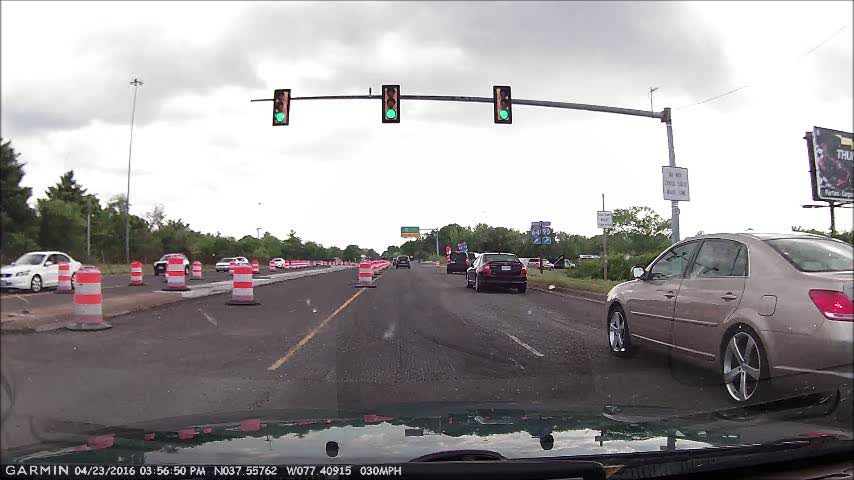The image, timestamped "Garmin 04-23-2016, 3:56:50 pm" and displaying a speed of 30 miles per hour, appears to be captured from the hood of a car, as seen through the windshield. This car is positioned in the left-hand lane of a multi-lane road approaching a traffic light, which is green, indicating that vehicles can proceed. Ahead, several vehicles are visible in both the left and right lanes, with the majority in the right lane preparing to turn right. Oncoming traffic is visible on the opposite side of the road, predominantly consisting of white cars. The scene includes heavy-duty pylons placed in the median and partially on the road. In the background, there is a billboard along with various road signs, although the text on these signs is too distant to be legible.